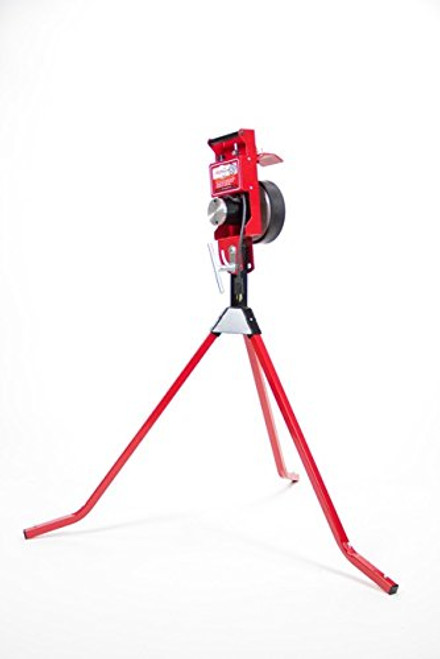In this image, the focal point is a single surveying device positioned centrally against a completely white background. The device stands on a tripod with three metallic legs, likely made of aluminum, that spread downward towards the bottom corners of the image, providing stability to the equipment. The tripod legs converge at a black joint, above which sits the main apparatus. 

The upper portion of the tool is a vibrant red and features several distinct elements. On the side, there's a lens with a black cap, along with a silver dial positioned towards the front. The legs and various components are colored in shades of gray, black, red, and silver. The setup and presentation suggest the image was perhaps taken for a product listing, possibly for sale in a home improvement store.